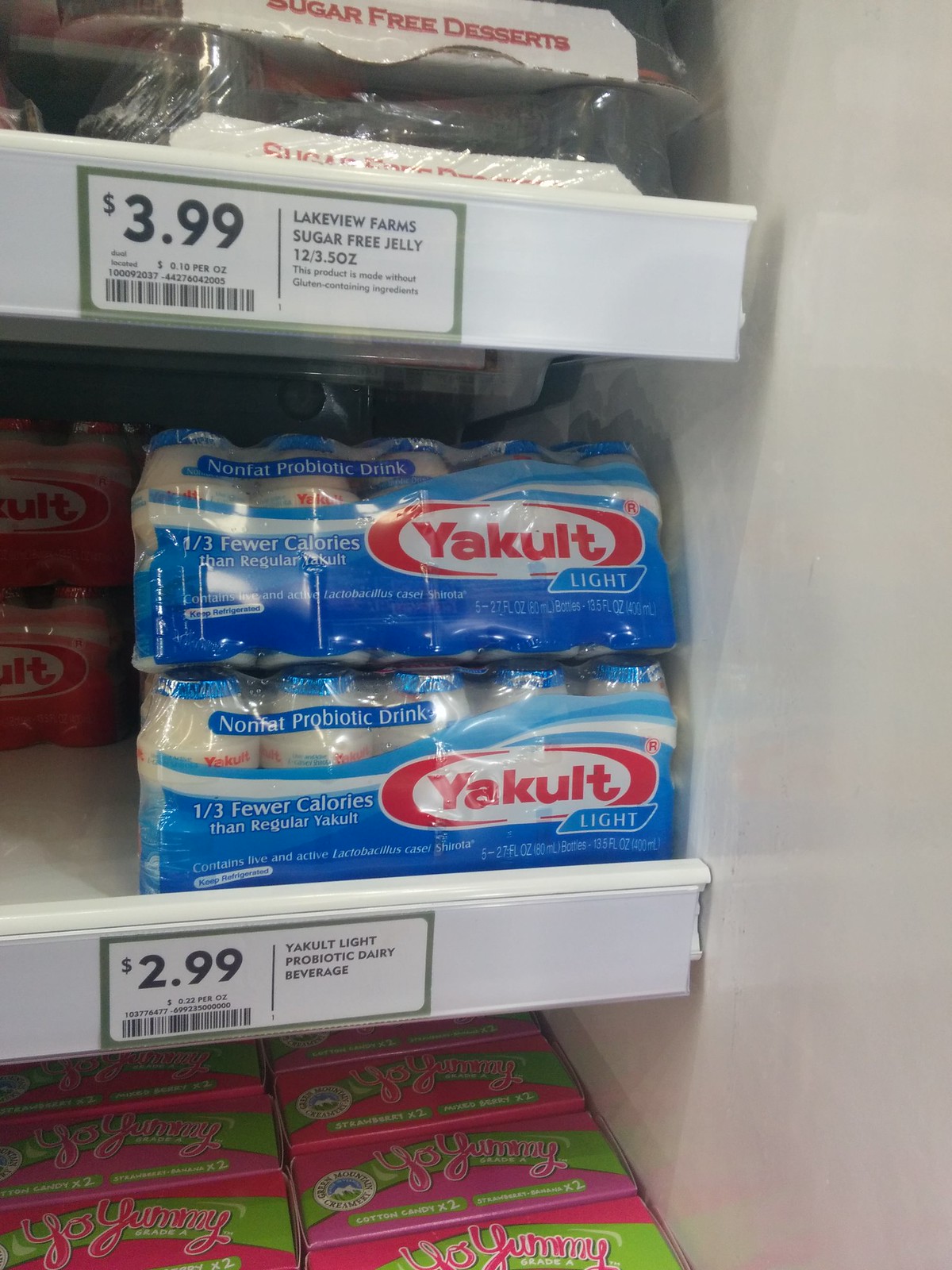The vertically-oriented color photograph captures three shelves in a grocery or convenience store. The top shelf displays two packages wrapped in cellophane labeled "Lakeview Farms Sugar-Free Jelly" priced at $3.99, with a sign indicating they come in 12 packs of 3.5 ounces. The packages bear the word "Sugar-Free Desserts" in white text on red backgrounds. The middle shelf shows "Yakult Light Probiotic Dairy Beverage" priced at $2.99. The blue and white packaging states, "1/3 fewer calories than regular Yakult" and "Nonfat Probiotic Drink." In the background, a red variant of Yakult can be seen, presumably the regular version. The bottom shelf contains boxes labeled "Yo Yummy" in a stripe across the top, available in flavors such as Cotton Candy and Mixed Berry, with no visible price tag. The scene captures a variety of probiotic drinks and dairy-related products, emphasizing their health benefits like aiding digestion and supporting the immune system.